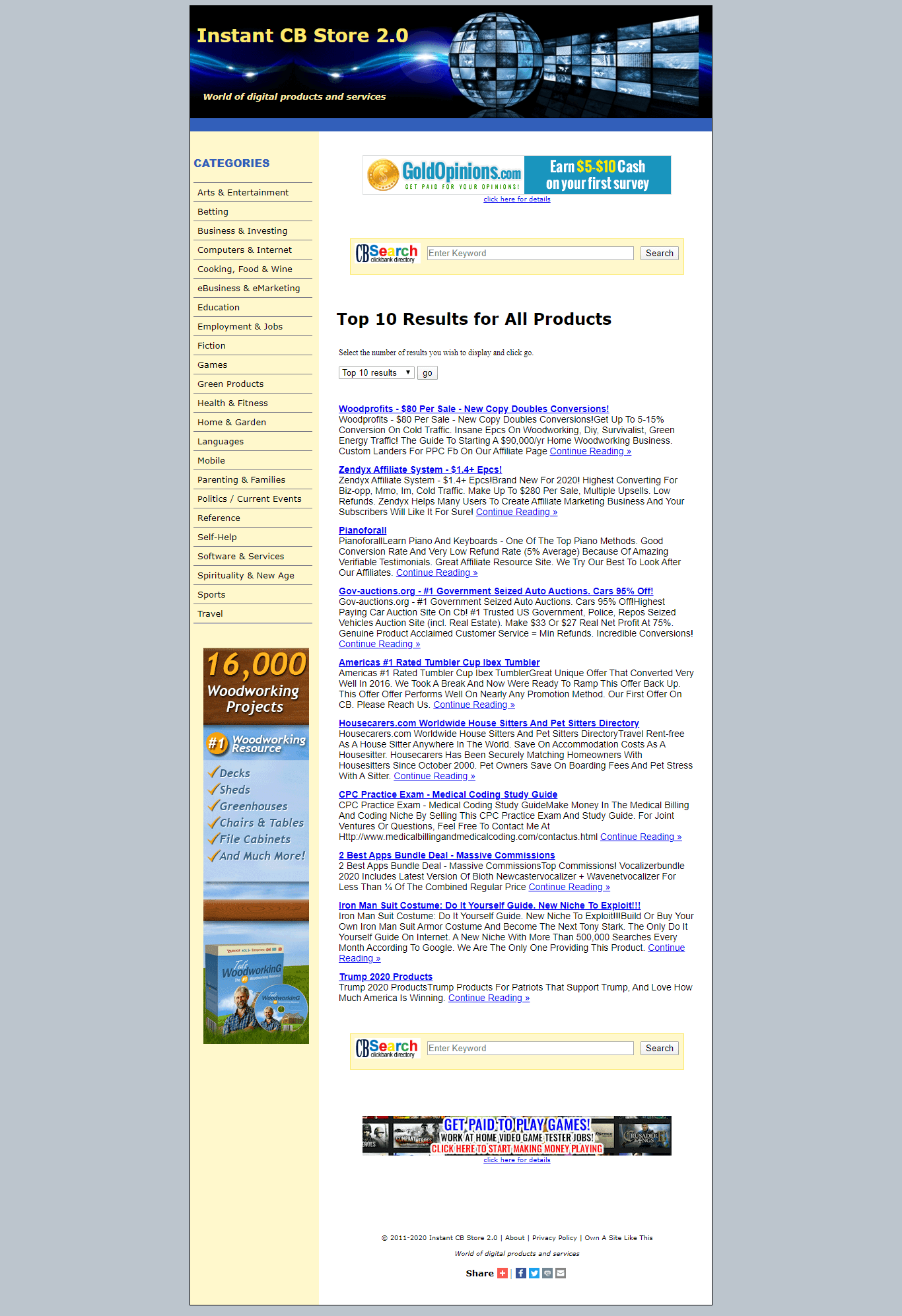The image depicts a full-page capture of a website with a solid light grey background. The website header prominently features the title "InstantCBStore2.0" accompanied by a circular logo containing multiple monitor icons. Adjacent to the logo, there is a banner with angled monitors set against a black background accented by a blue wave design and yellow text beneath it.

On the left side of the webpage, there is a light yellow section labeled "Categories" in blue text, followed by several unreadable subsections. Below this, there is a media image advertising "6,000 Woodworking Projects" with accompanying details about the offer.

The main content area includes an advertisement from "goldopinions.com" announcing an opportunity to earn between $5 to $10, positioned above a search bar labeled "Search." Below the search bar, a list titled "Top 10 Results for All Products" is displayed, with each product title highlighted in blue font.

At the bottom of the page, there is an additional advertisement promoting "Get Paid to Play Games."